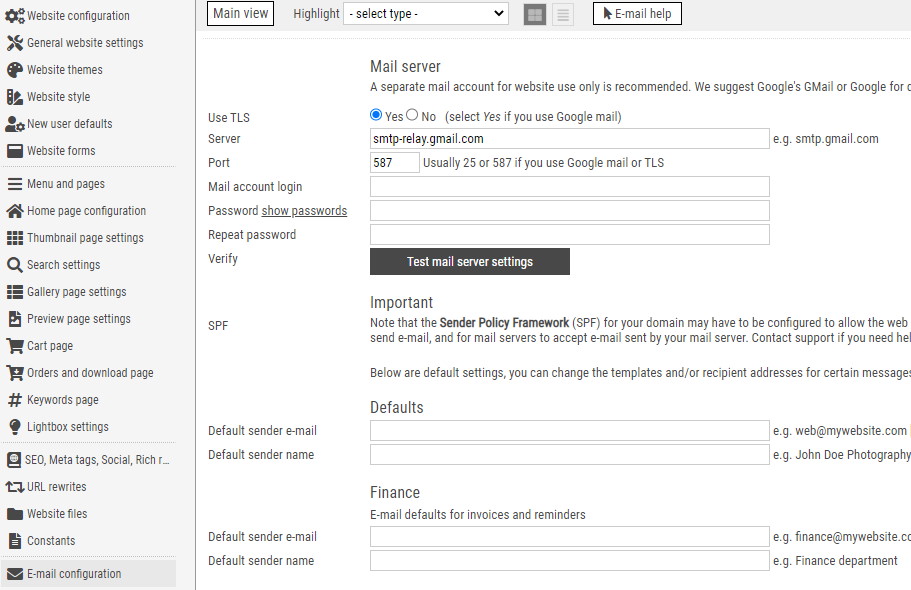**Detailed Screenshot Caption of an Email Configuration Dashboard:**

The image depicts a comprehensive screenshot of a dashboard designed for email or website configuration, resembling the interface of a content management system such as WordPress. The left-hand side features an extensive side menu with numerous navigable options, including "Website Configuration," "General Website Settings," "Website Themes," "Website Style," "Menu and Pages," "Homepage Configuration," "Thumbnail Settings," "Search Settings," "Gallery Settings," "Preview Settings," "Cart Page," "Order and Download Page," "Keyword Page," "Lightbox Settings," "SEO Meta Tags," "URL Rewrites," "Website Files," "Constants," and "Email Configuration." The "Email Configuration" option is currently highlighted, indicating the active section being viewed.

The main view is set against a clean white background adorned with black text. This section contains various input fields, some pre-filled and others left blank. At the top of this view, the heading "Main View" is prominent, accompanied by options such as "Highlight," "Select Type" (a dropdown menu), and "Email Help."

The focal point of this section is the "Mail Server" configuration, which is tasked with setting up a separate mail account recommended exclusively for website use. Suggested services include Google Mail (Gmail) or Google-related options. There is a toggle for "Use TLS," which is currently set to "Yes," with a note clarifying that this should be selected if using Google Mail. The SMTP server address is specified as "smtp-relay.gmail.com," and the port number is designated as "587."

Subsequent fields for "Mail Account Login," "Password," "Repeat Password," and "Verify" remain blank, ready for input. A notable section labeled "Important" urges users to configure the Sender Policy Framework (SPF) for their domain to authorize the website to send emails.

Additional settings include defaults for the "Default Sender Email Name," "Email," and "Email Name." There is also a specified default for finance-related emails, labeled "Default Sender Email Name for Finance."

Overall, this screenshot captures the intricate details of a website's email configuration page, underscoring the meticulous setup required for efficient email communication management.